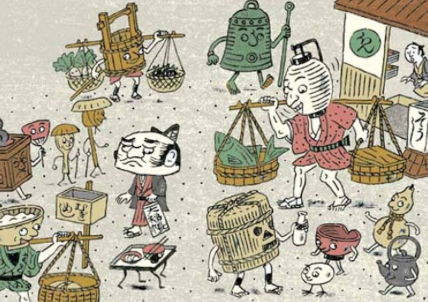This image is a vibrant and whimsical drawing featuring various animated cartoon characters. At the forefront is a green character shaped like the top of a bell, complete with tiny arms and legs. Another character is energetically carrying a pole with a basket of fish and an empty basket attached. To the side, there is a small gray walking teapot and a lively pink cup, both miraculously brought to life and parading around. Among these playful figures stands a grumpy-looking, bald-headed man with an oversized head, dressed in a pink dress and purple jacket, adding a touch of eccentricity to the scene. In the background, a building captures attention with a figure resembling a Japanese man peering through the doorway, adding a cultural layer to the dynamic composition. The entire image exudes an imaginative and animated atmosphere.